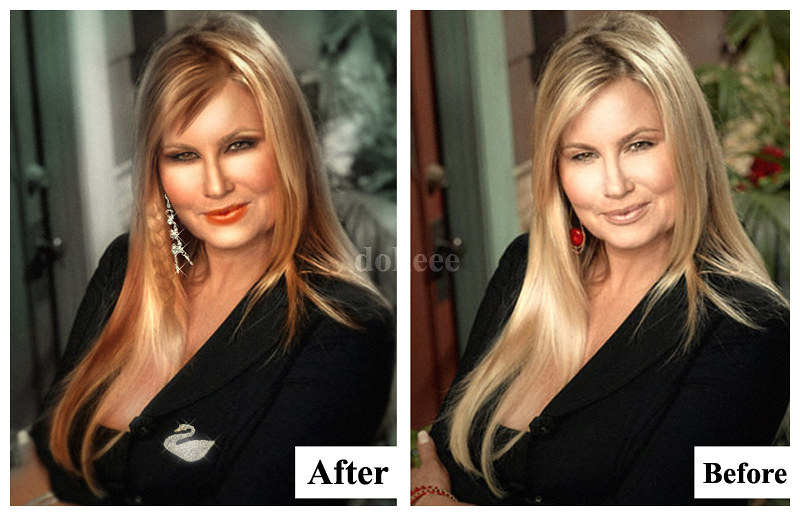The image is a side-by-side comparison of two photographs of the same woman, showing the before and after effects of digital enhancements. The photograph on the right, labeled "before" at the bottom right in a white rectangle with black text, features the woman facing forward and smiling slightly. She is a white female with dyed blonde hair, wearing a black business coat over a low neckline black shirt, and sporting red earrings. Behind her is a floral arrangement consisting of white and red flowers with green leaves. The photograph on the left, labeled "after," depicts the digitally enhanced version of the same image. In this edited photograph, her makeup has been intensified, and her earrings have been swapped out for dangling diamond ones. Additionally, a small pin resembling a swan is visible on her jacket, and the overall hue has been altered to give a slightly computer-generated appearance. The enhancements also amplify her features, giving the photograph a more polished and stylized look. Both photographs are separated by a solid white line down the middle, clearly highlighting the differences between the natural and enhanced versions. The woman's shoulders are angled slightly to the left, and although part of her hand with some bracelets can be seen at the bottom left of the "before" image, it is not prominent in the "after" photograph. The setting appears to be indoors, though the time of day is indeterminate.